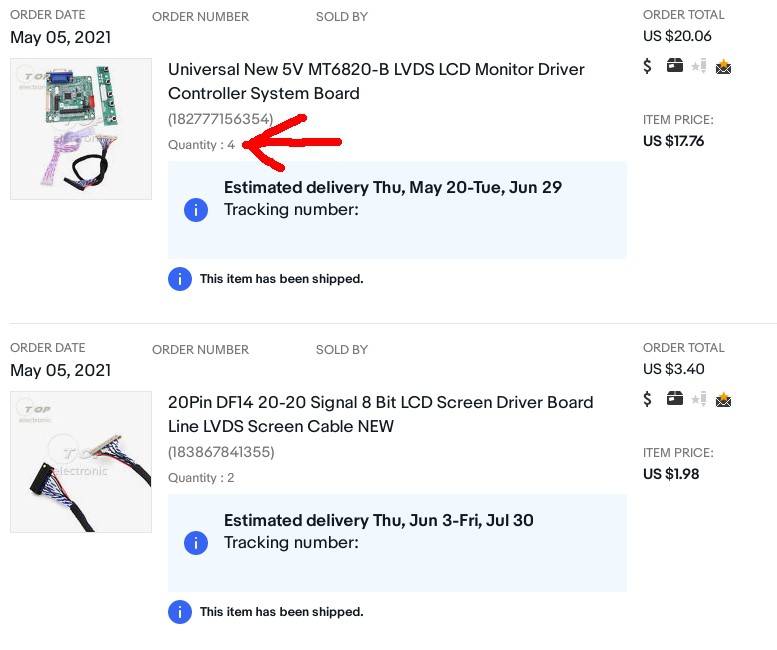This image is a screenshot from an e-commerce website, likely eBay given its characteristic layout, with a white background. The screenshot is taken from a user's order section within their account. A red arrow has been added to the image, pointing specifically to the quantity number of a purchased product.

In the screenshot, there are two ordered products visible, stacked vertically. The top product, which the red arrow highlights, has the following details: 
- Order date: May 5, 2021
- Description: Universal New 5V MT6820-B LVDS LCD Monitor Driver Controller System Board
- Quantity: 4 (emphasized by the red arrow)
- Item cost: $17.76
- Total cost including tax and shipping: $20.06
- Estimated delivery: Thursday, May 20 through Tuesday, June 29

Additionally, there's an accompanying image of some computer components next to the product description. This detailed breakdown underscores the primary focus of the screenshot — the quantity of the ordered item, accentuated by the red arrow.